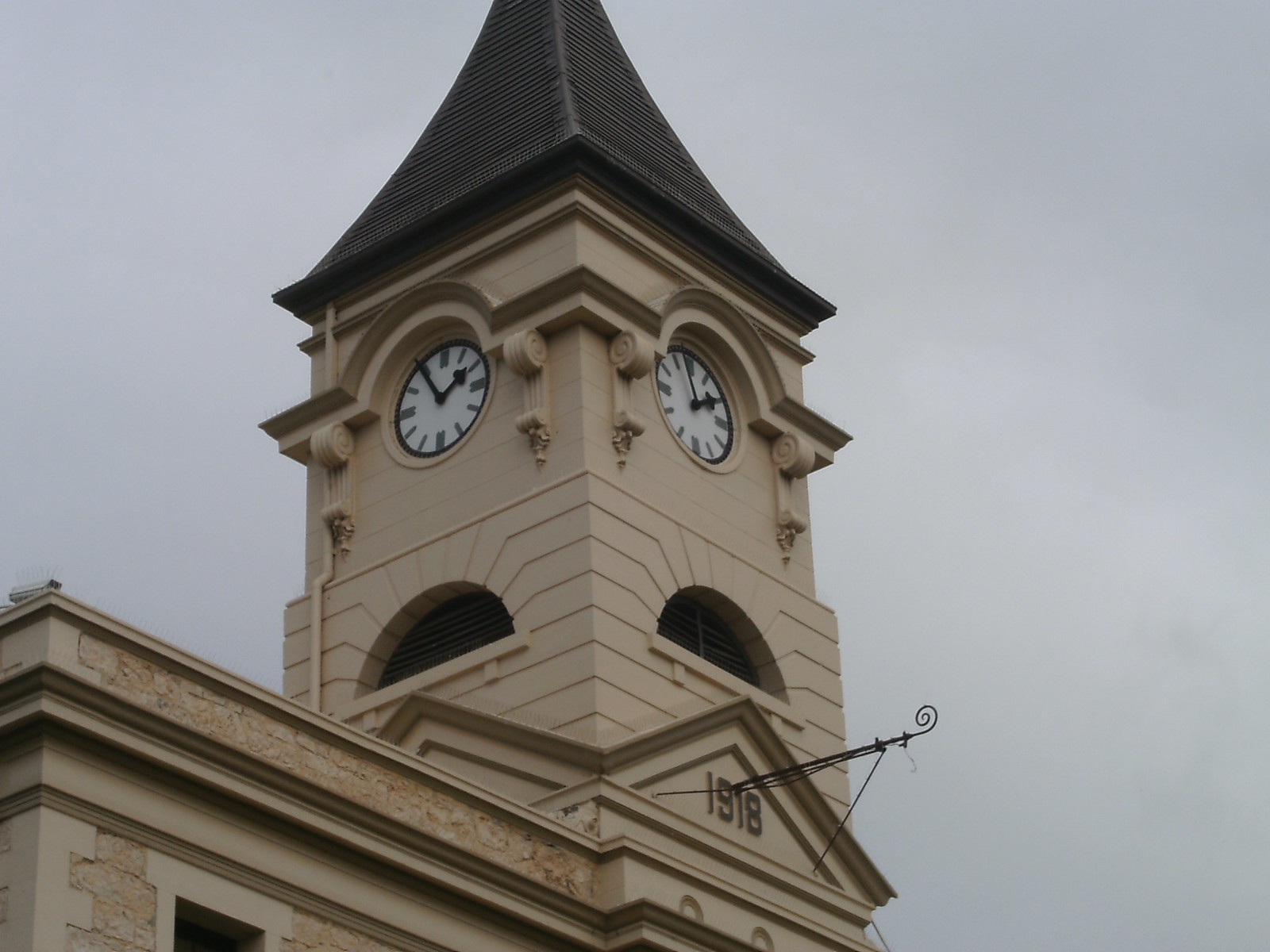The photograph captures an outdoor scene featuring the prominent corner of a historic building with a clock tower. The image is taken from the ground, looking up at the structure. The tower, which rises from the rectangular building, has a dark brown or black triangular, pointy roof. Below this roof, there's a square section with a circular clock on each visible side, both featuring black Roman numerals and hands. The clocks display a time close to 1:55. The upper part of the tower has strong architectural arches and open lookouts, giving it an ornate appearance. The building itself is tan or light brown and has the year "1918" inscribed on the front, possibly indicating the year of its construction. Extending from the building's left side is a visible ledge that supports a security camera. The sky in the background appears overcast, with varying shades of gray, lending a muted tone to the photograph.